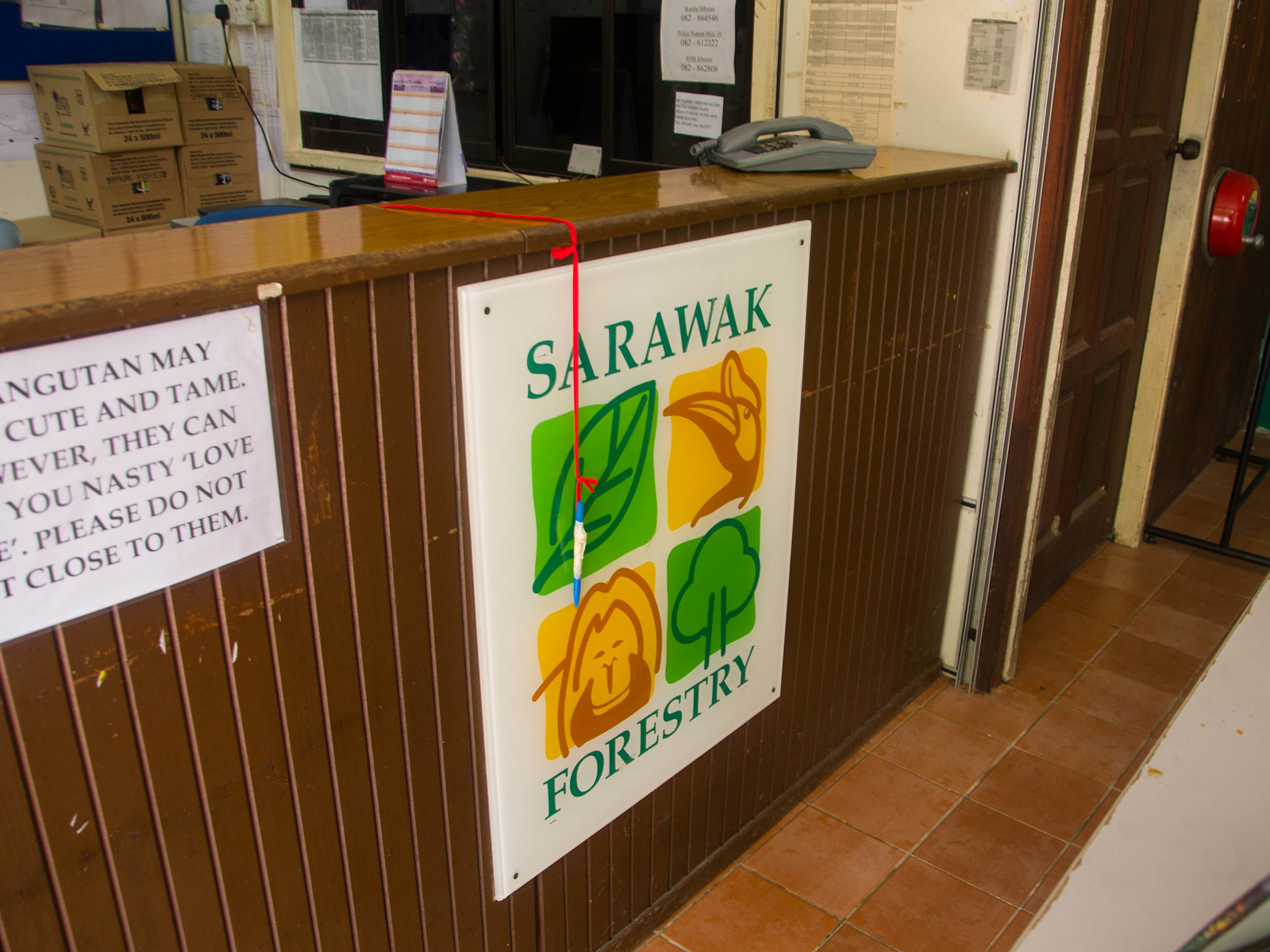The image depicts the interior of an office or service counter, likely related to the Sarawak Forestry in Indonesia or a similar region. The primary focus is a brown stand with a white sign on its front. Prominently displayed on the sign are the words "Sarawak" at the top and "Forestry" at the bottom, with green typography. Centrally, the sign features four square images: a green leaf in the top left, a yellow monkey in the bottom left, a yellow bird in the top right, and a green tree in the bottom right.

On top of the brown countertop, there's an old-fashioned dial telephone, adding a nostalgic touch to the setting. A pen attached to a red string dangles from the stand, suggesting it is meant for visitors to use, potentially to sign in or fill out forms. The environment implies it is dedicated to conservation efforts, possibly for orangutans, as indicated by a partially visible warning about interactions with the animals. Additional context in the image includes some boxes on the upper left of the stand and a door to the right, extending beyond the counter's end.